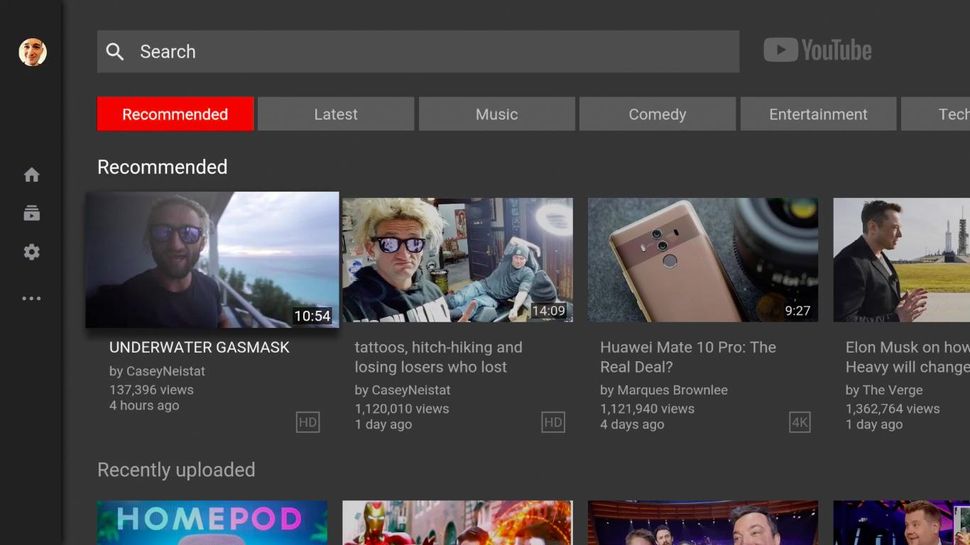A screenshot of the YouTube web page shows a partial view focused on the user's profile area and video recommendations. On the left side of the screen, there's a photograph of a young man smiling, serving as his profile picture. This is part of his YouTube page. Below the profile image, there are icons representing home, videos, settings, and a more options menu denoted by three horizontal dots. 

At the top of the page, the YouTube logo is positioned to the right of a search bar. Underneath, a highlighted red tab indicates the "Recommended" section, with adjacent tabs for "Latest," "Music," "Comedy," "Entertainment," and "Tech." Within the "Recommended" section, several video thumbnails are displayed, featuring diverse content such as an underwater gas mask tutorial, tattoos, hitchhiking tips, and a video titled "Losing Losers Who Lost." Additionally, there are other videos like a review of the Huawei Mate 10 Pro smartphone, and an incomplete title mentioning Elon Musk.

Further down, in the "Recently Updated" section, only parts of the video titles are visible. One mentions the HomePod, another appears to be a Marvel-related video, one might feature Stephen Colbert, and another points to various entertainment topics focusing on actors.